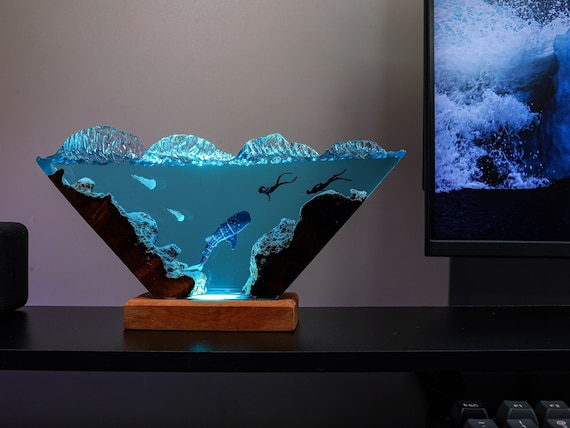The image captures a fascinating decorative piece in a home's interior. Dominating the scene is a black shelf on the left, with a flat-screen TV partially visible on the right side, displaying dynamic visuals, possibly involving water. Central to the composition sits a striking light fixture resembling an aquarium but crafted from epoxy resin. This light has a wooden base and rises in an inverted pyramid or V-shape, filled with vivid blue resin mimicking an underwater scene. Immersed within this resin are intricate details including a miniature whale, a couple of jellyfish, and the silhouettes of divers, all suspended as if in mid-swim. The resin’s surface is textured to emulate ocean waves, and the base of the fixture is illuminated, drawing attention to the artistic depiction of an underwater rock trench. On the far left of the shelf, a small, indistinguishable black box subtly adds to the scene's depth. The piece is an eye-catching blend of art and light that instantly captivates viewers.